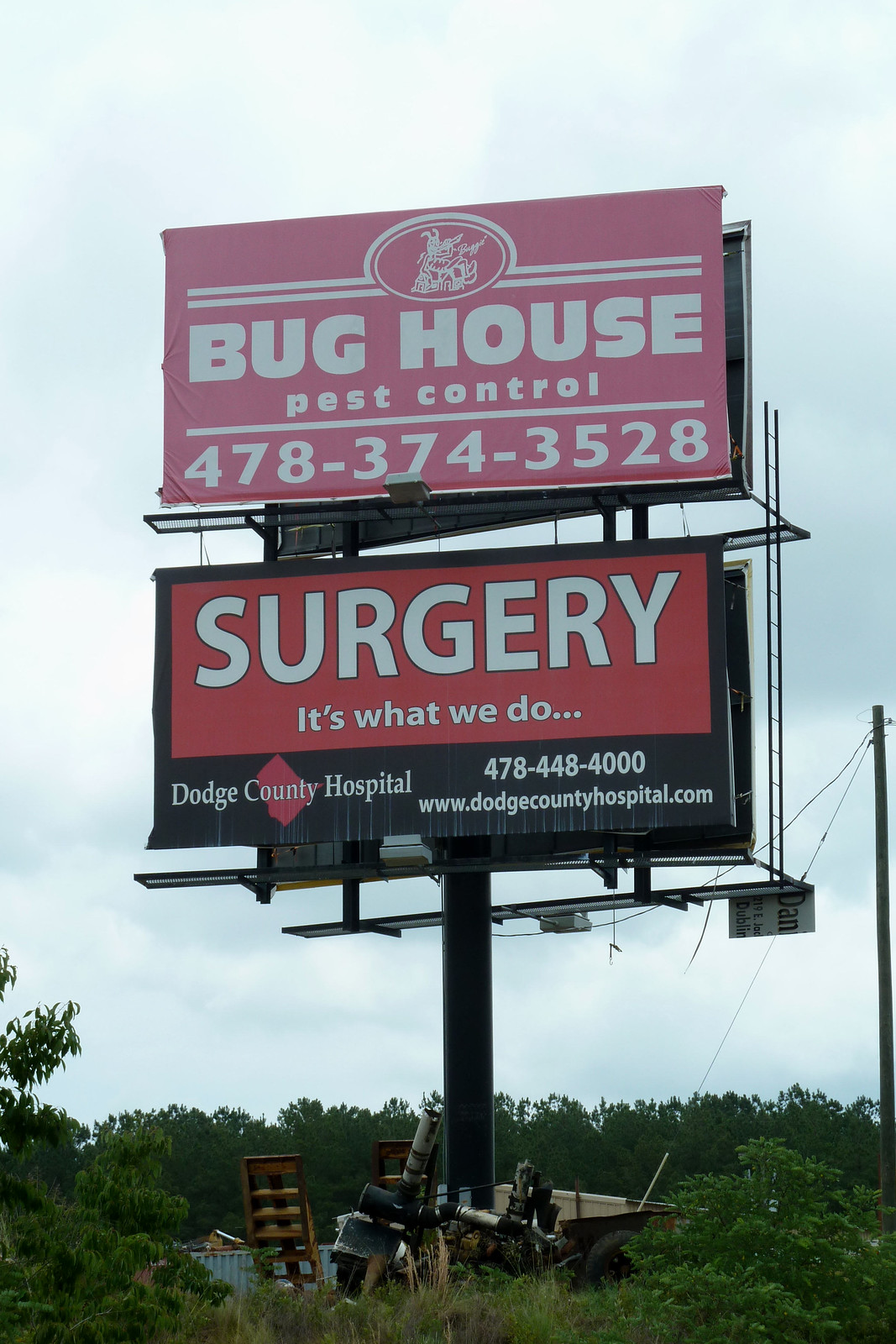The image is a detailed, vertically oriented color photograph showcasing two large billboards mounted on a single black metal pole, set against a backdrop of a partly cloudy sky with patches of bright white and light blue. Surrounding the pole and filling the foreground are various pieces of metal clutter, large wooden items such as pallets or steps, and lush green foliage, including trees and bushes. In the distance, tall green trees form a forested area.

The top billboard features a light red background with a logo of a bug encircled at the top, flanked by two lines. Prominently displayed in white capital letters are the words "BUG HOUSE," with "Pest Control" written below in smaller lowercase letters and a dividing line under it. A 10-digit phone number "478-374-3528" is also included.

Below it, the bottom billboard has a black background with a large inner rectangle shaded medium red occupying its top two-thirds. Inside this rectangle, the word "SURGERY" is written in bold white capital letters, with the phrase "it's what we do" in smaller white letters beneath it. Further down on the black background, in the lower-left corner, "Dodge County Hospital" is displayed along with a phone number "478-488-400" and a website URL, both in white text.

This structured scene effectively highlights the two distinct advertisements, their supportive framework, and the natural elements surrounding the display.